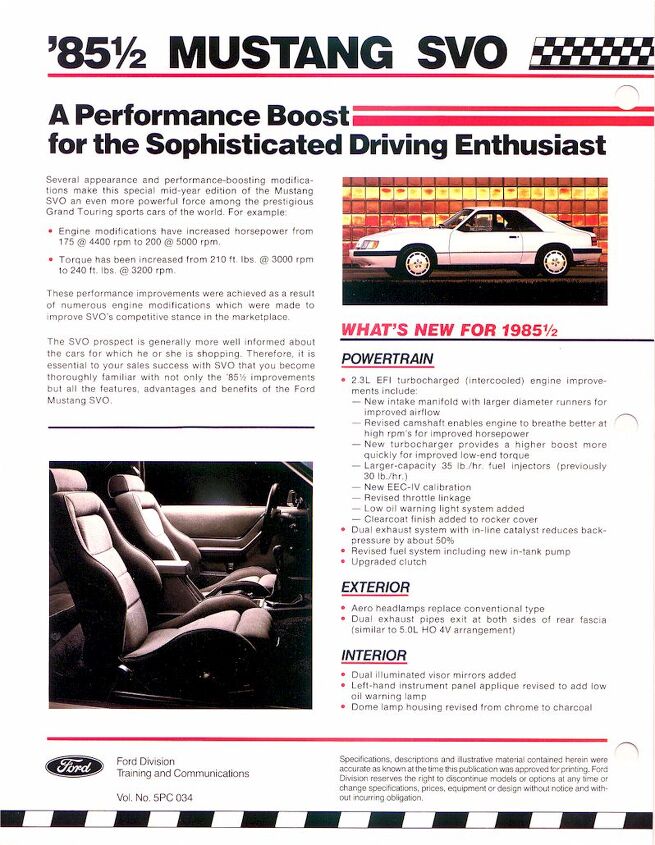This image, oriented in portrait and possibly taken from a car spec binder, showcases an advertisement for the 1985.5 Mustang SVO. The title reads "85.5 Mustang SVO" in black text at the top, followed by a black and white checkered racing banner and a red line. Underneath, it states, "A performance boost for the sophisticated driving enthusiast." The ad highlights several appearance and performance modifications that make this mid-year edition of the Mustang SVO even more powerful. The improvements are detailed in a paragraph on the left, explaining engine modifications that increased horsepower from 175 at 4,400 rpm to 200 at 5,000 rpm, and torque from 210 foot-pounds at 3,000 rpm to 240 foot-pounds at 3,200 rpm. The ad emphasizes the importance of understanding these enhancements for sales success. 

On the right, there's a picture of a white Mustang, captured outdoors and facing left, with accompanying text broken down into sections on "Powertrain," "Exterior," and "Interior" details. Additionally, there is a photo of the Mustang’s interior, showing bucket seats, in the bottom left corner, and the text "Ford Division Training and Communications, Volume Number 5 PC 034" at the bottom. The detailed design and layout suggest a sophisticated and well-informed target audience for this sporty and improved Mustang model.